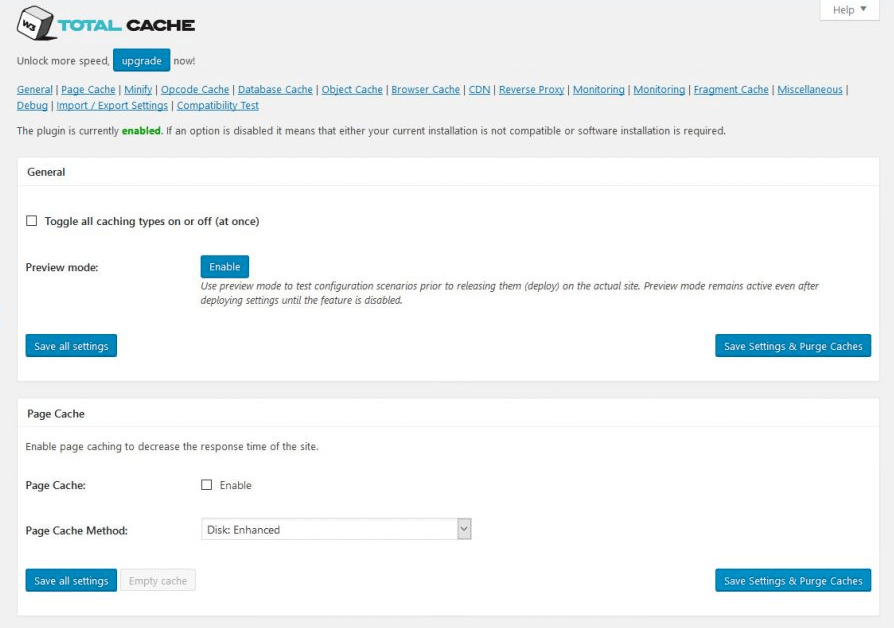This image appears to be a screenshot of the Total Cache plugin settings page for a website. The "Total Cache" heading features "TOTAL" in blue letters and "CACHE" in black letters. To the left, there's a cube icon with "W3" inside.

Beneath the main heading, a message reads, "Unlock More Speed, Upgrade Now," with the "Upgrade" option highlighted in blue, indicating a clickable button.

A navigation menu is displayed below the heading, including the following options:
- General
- Page Cache
- Minify
- Opcode Cache
- Database Cache
- Object Cache
- Browser Cache
- CDN (in capital letters)
- Reverse Proxy
- Monitoring
- Fragment Cache
- Miscellaneous
- Debug
- Import/Export Settings
- Compatibility Test

The interface indicates that the plugin is currently enabled, with the word "enabled" highlighted in green. A note mentions that if an option is disabled, it may be due to incompatibilities or missing software installations.

The "General" settings section features a white box with an unchecked option labeled "Toggle All Caching Types On or Off at Once." Below this, there's an option for "Preview Mode" with a blue "Enable" button, accompanied by an explanation that preview mode allows users to test configuration scenarios before deploying them on the actual site. It emphasizes that preview mode remains active even after settings are displayed until the feature is disabled.

At the bottom of the General section, there are two blue buttons: "Save All Settings" on the left, and "Save Settings and Purge Caches" on the right.

Further down, the "Page Cache" section includes an explanation that enables page caching to decrease the site's response time. There is an unchecked "Enable" box, and a "Page Cache Method" drop-down menu showing "Disk: Enhanced" as the selected option. Below this section, there are two buttons related to cache management: "Save All Settings" in blue on the left, and "Empty Cache" grayed out. Lastly, on the far right, there is a blue "Save Settings and Purge Caches" button.